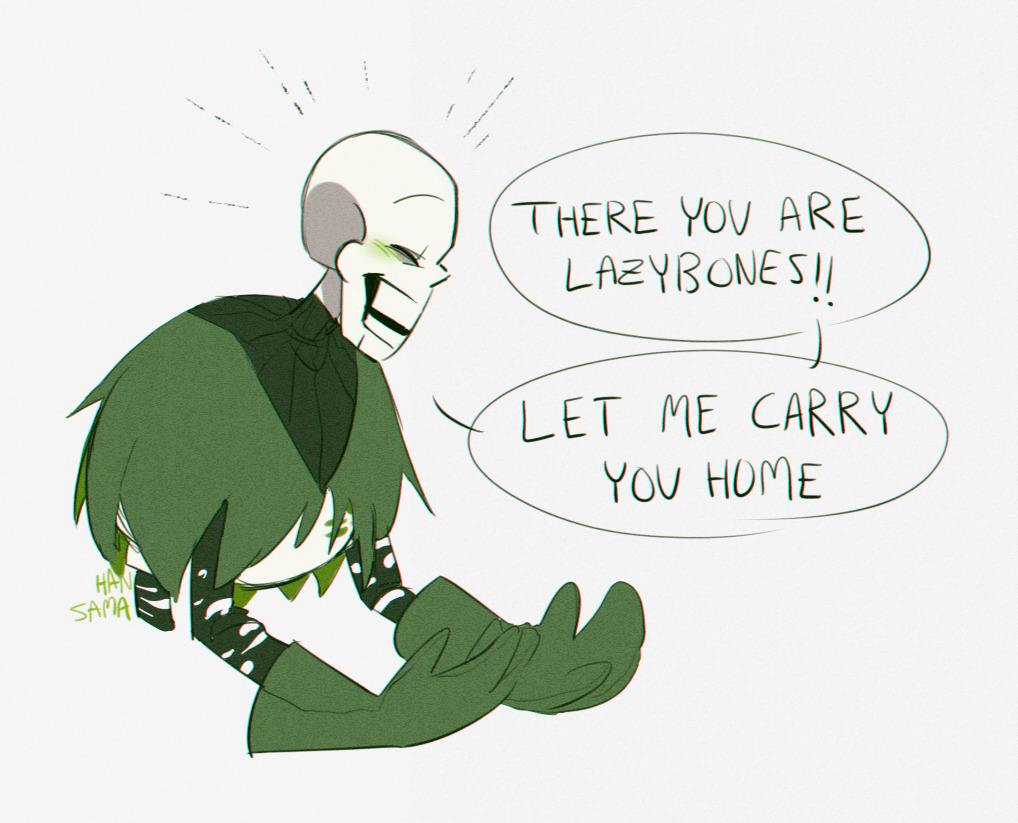A detailed comic-style illustration against a white background features a skeleton-faced character on the left, shown in profile view, facing to the right with an exasperated expression. The character has a white skull head with a faint green blush around the eye, highlighted by a few straight lines emanating from the head to indicate emotion. The skeleton wears a ripped green short cap, a matching green long-sleeve overcoat, a green and white polka-dotted shirt underneath, a white chest plate, and large green gloves. Below the figure is the word "HANSAM" printed or written in green. On the right side of the image are two speech bubbles with black text. The top bubble reads, "There you are, lazy bones," and the bottom bubble says, "Let me carry you home."